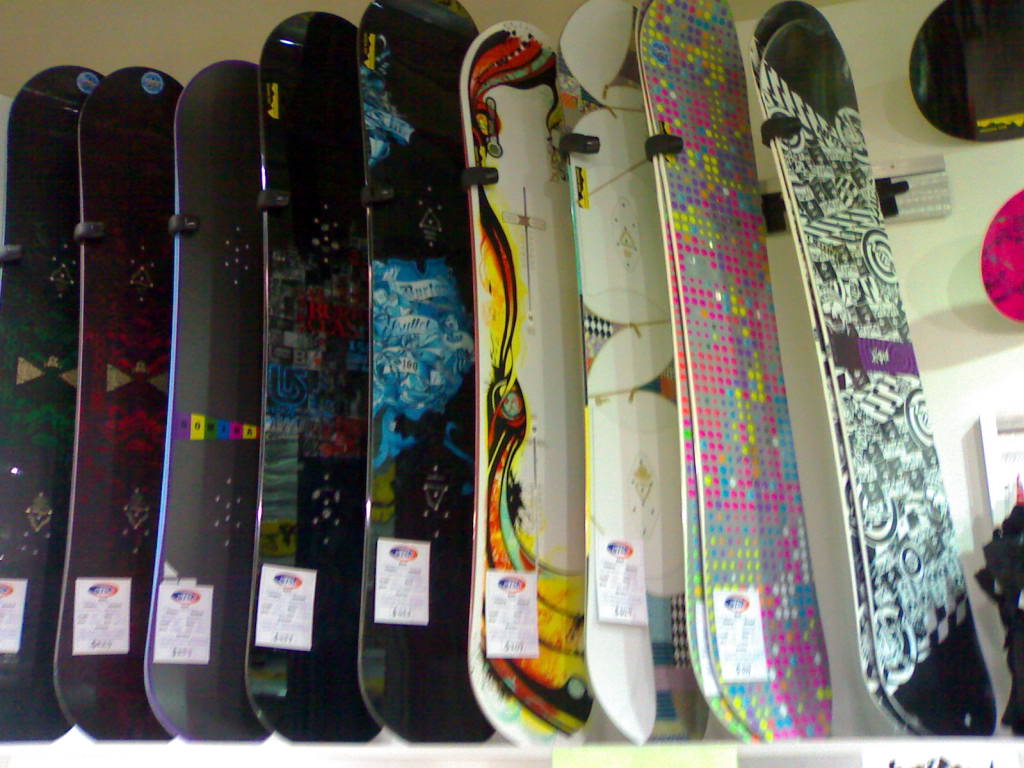In the image taken inside a shop, a pristine white wall serves as the backdrop for a vibrant display of snowboards mounted on the wall with clasps. The showcases feature a diverse array of colors and patterns, creating a striking visual spectacle. Nine snowboards are neatly aligned horizontally, with two additional snowboards partially visible in the top right corner.

The first five snowboards, each adorned with unique designs, share a predominantly black base. The first two have face designs, colored green and red, respectively. The next is purely black with no other designs. The fourth features a quilted mosaic pattern of different colors and lettering, resembling a xylophone. The fifth snowboard bears cursive writing and numbers intertwined with blue and white ribbon-like patterns.

Adjacent to these, a snowboard with a flaming Inferno design transitions from yellow at the base to black towards the top. The next snowboard, featuring a diamond checker pattern and crisscross squares, is based in white. The following pink snowboard is decorated with a playful assortment of squares in yellow, pink, white, and blue. Finally, the display is anchored by a snowboard with a dynamic black-and-white graffiti design on the far right.

Each snowboard, except for the far-right one, has a piece of paper attached, likely indicating the price. Although the labels are blurry and the logos are indiscernible, the overall scene captures a colorful and energetic display of snowboarding gear.